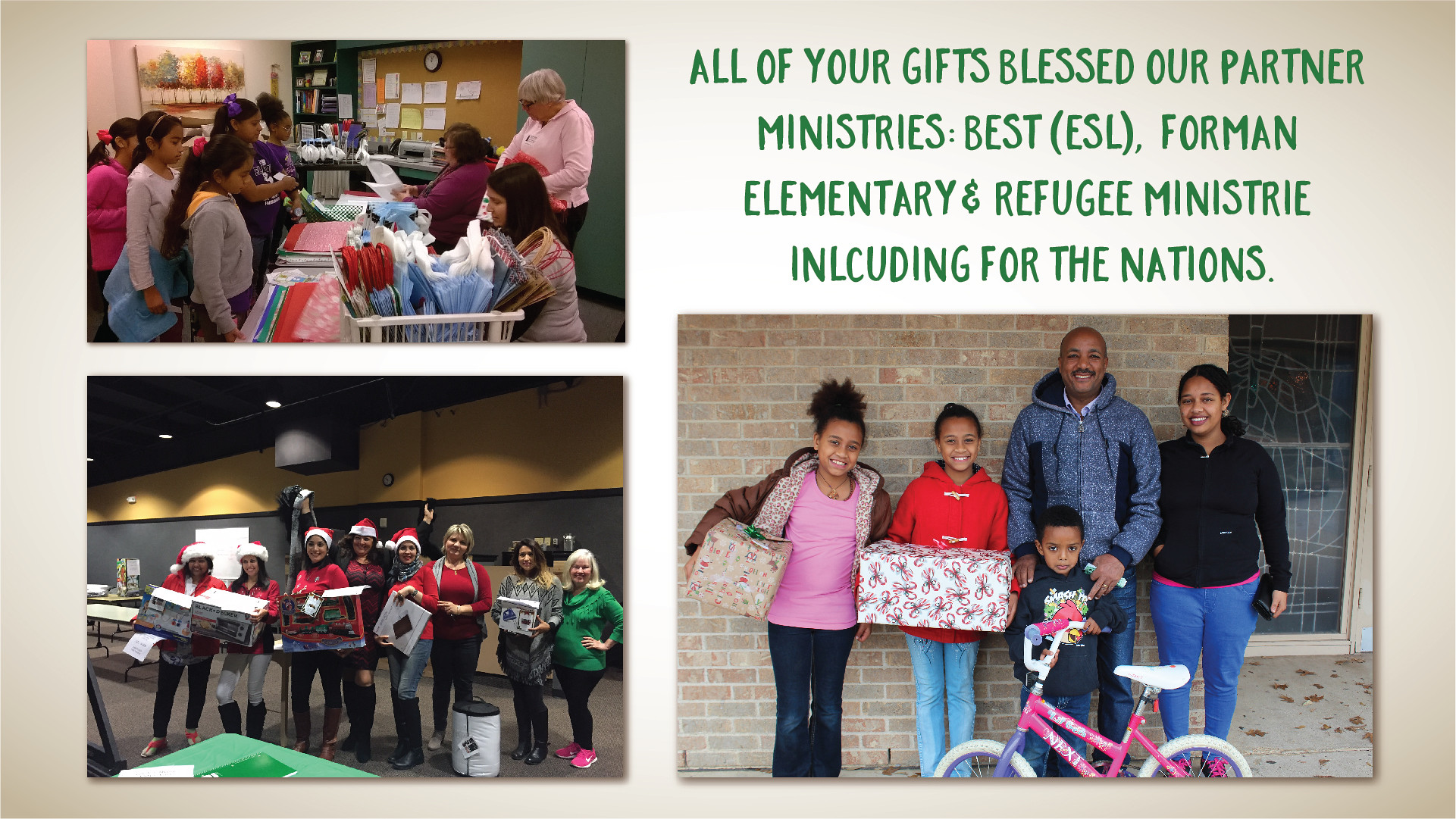This wide rectangular digital collage has an off-white background that transitions to gray at the edges. In the top right corner, a green caption reads, "All of your gifts blessed our partner ministries: Best ESL, Foreman Elementary, and Refugee Ministry, including For the Nations." This image is comprised of three main photos:

1. **Top Left Photo**: A group of young girls stands behind a registration desk where women in pink and red are seated, suggesting a charity or event registration.
2. **Bottom Left Photo**: A gathering of volunteers dressed in festive Christmas attire, including Santa hats, all smiling and holding boxed gifts, symbolizing holiday spirit and generosity.
3. **Bottom Right Photo**: A joyful family of five, including a man, a woman, and three children, proudly displaying Christmas presents they received, reflecting the positive impact of the gift drive.

These photos collectively illustrate a holiday charity event where gifts were distributed to communities supported by partner ministries, highlighting the collaborative and festive nature of the occasion.